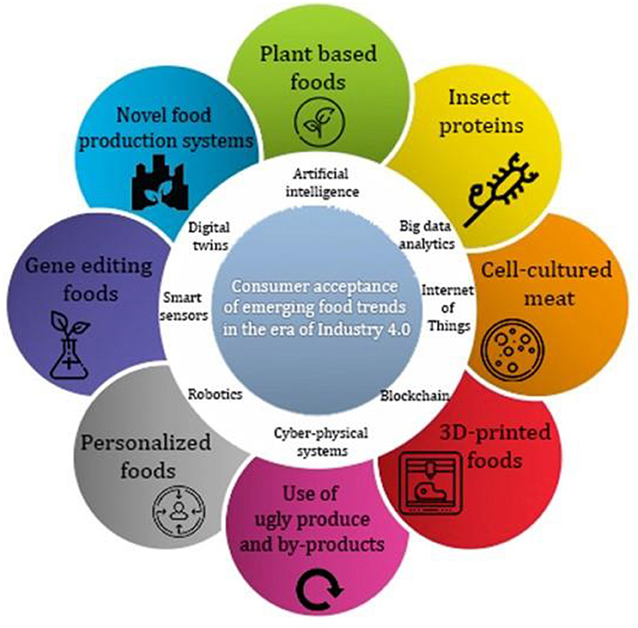The image is a detailed circular diagram centered around "Consumer Acceptance of Emerging Food Trends in the Era of Industry 4.0" highlighted in bold white lettering on a blue central circle. Surrounding this central circle is a white ring with black text listing key technological themes: Artificial Intelligence, Big Data Analytics, Internet of Things, Blockchain, Cyber Physical Systems, Robotics, Smart Sensors, and Digital Twins. Encompassing this white ring are eight vividly colored circles, each representing different food innovations. These include olive green for Plant-based Foods, yellow for Insect Proteins with an insect outline, orange for Cell-cultured Meat, red for 3D Printed Foods, purplish-pink for Use of Ugly Produce and Byproducts, gray for Personalized Foods, purple for Gene Editing Foods, and blue for Novel Food Production Systems. The entire diagram emphasizes the integration of advanced technologies and novel food production methods in shaping the future of food trends.